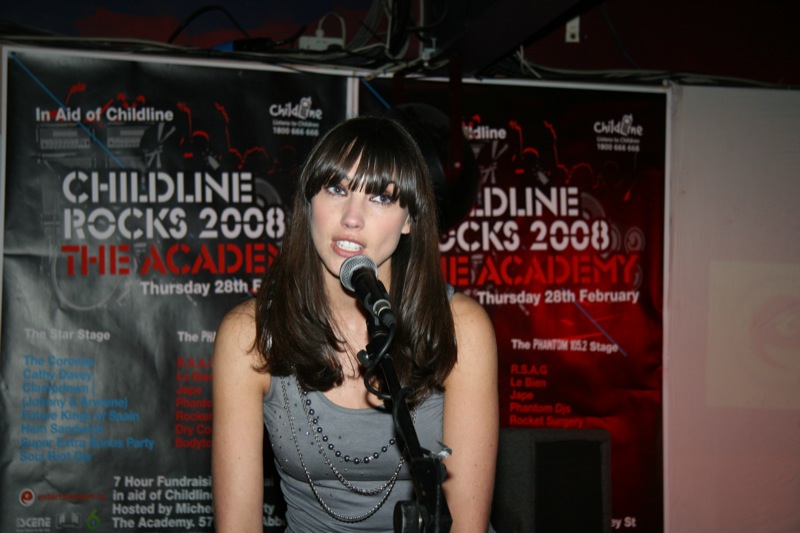The photograph captures a young woman in her early 20s, with long, dark brown shiny hair and bangs that reach just to the tops of her eyes, which are accentuated with mascara. She has light eyes and fair skin. She is slightly tilting her head to the left as she speaks into a microphone. She is wearing a gray tank top and several strands of long gray bead necklaces. The setting appears to be a stage, indicated by the lighting wires visible above her head and the presence of various cords and cables. 

Behind her is a large black poster with white text that reads, “In aid of Childline. Childline Rocks 2008. The Academy. Thursday 28th, February.” Although her position obscures part of the poster, it mentions a seven-hour fundraiser hosted by a person named Mike, and two stage lineups with different bands are listed below the main text. This scene suggests a press conference or an announcement about the fundraiser event.